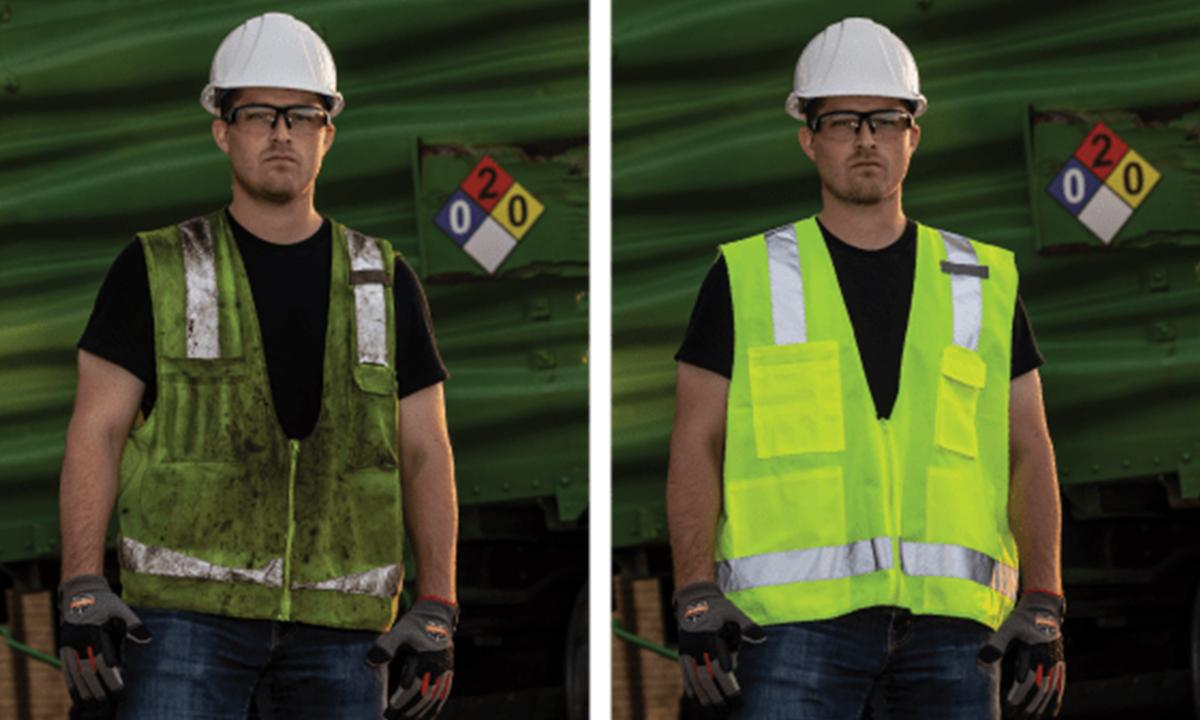This side-by-side comparison features a construction worker standing in the center of both photos. Both images capture the worker wearing identical outfits, consisting of a white hard hat, safety goggles, a black short-sleeve t-shirt, work gloves, denim jeans, and a yellow reflective vest. In the left photo, the worker's vest is extremely dirty, covered in mud and appearing very worn and tattered, with ripped reflectors. Contrastingly, the photo on the right shows the same worker in a spotless, clean vest that looks brand new. Both images share a green background, with a hazardous symbol appearing behind the worker's right shoulder, featuring the numbers "020" in a triangle with blue, red, and yellow sections. Despite the man being in the same stance, his appearance transitions from a day of hard work to a fresh start on the job.